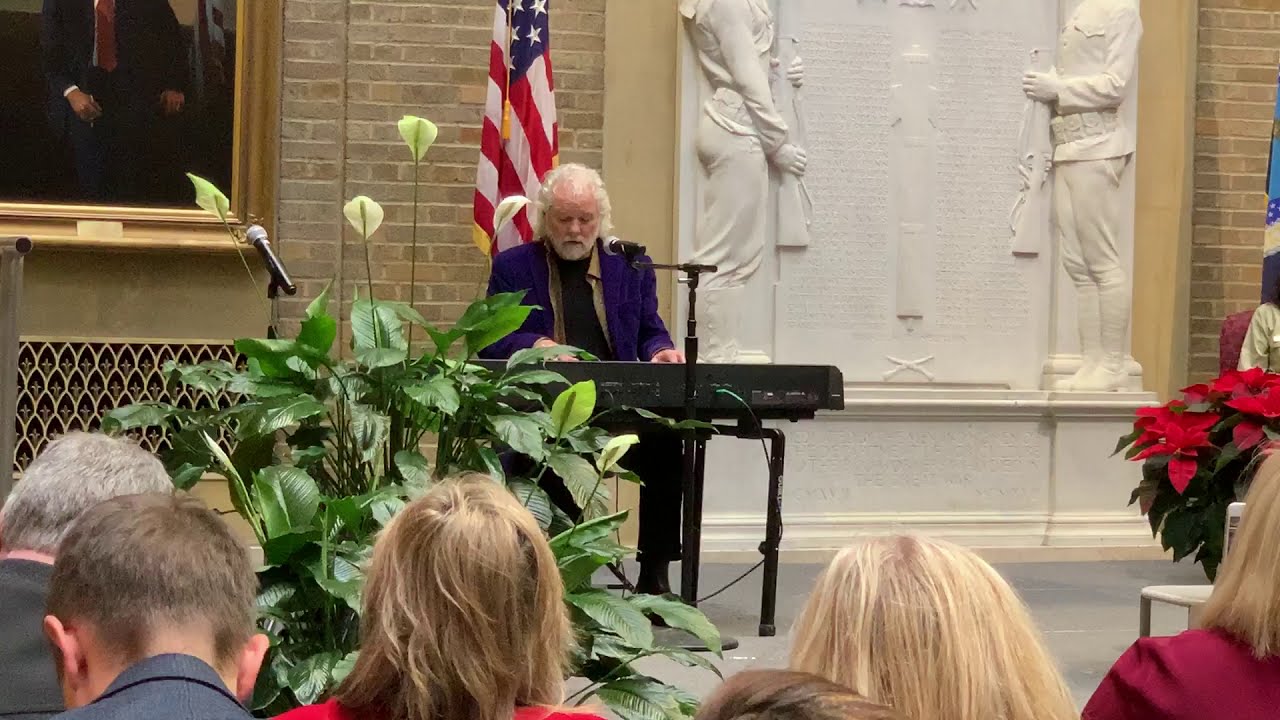In this image, a balding older man with long white hair, a white beard, and mustache is seated at a keyboard, positioned slightly left of center. He wears a dark purple jacket over an open brown collared shirt and a black undershirt. A microphone is positioned by his mouth, indicating he's singing or speaking as he plays. Directly in front of him, the heads of audience members with light-colored hair are visible, facing the stage. The backdrop features a variety of elements: a tan brick wall, an American flag, a large gold-framed painting to the left, and white relief sculptures depicting soldiers holding guns on the right. In the foreground, a healthy green plant with flowers is on the left and a poinsettia plant is on the right, adding vibrant touches of red and green to the scene. The overall setting suggests an indoor memorial service or a formal gathering, accentuated by the solemn decor and the central figure at the keyboard.